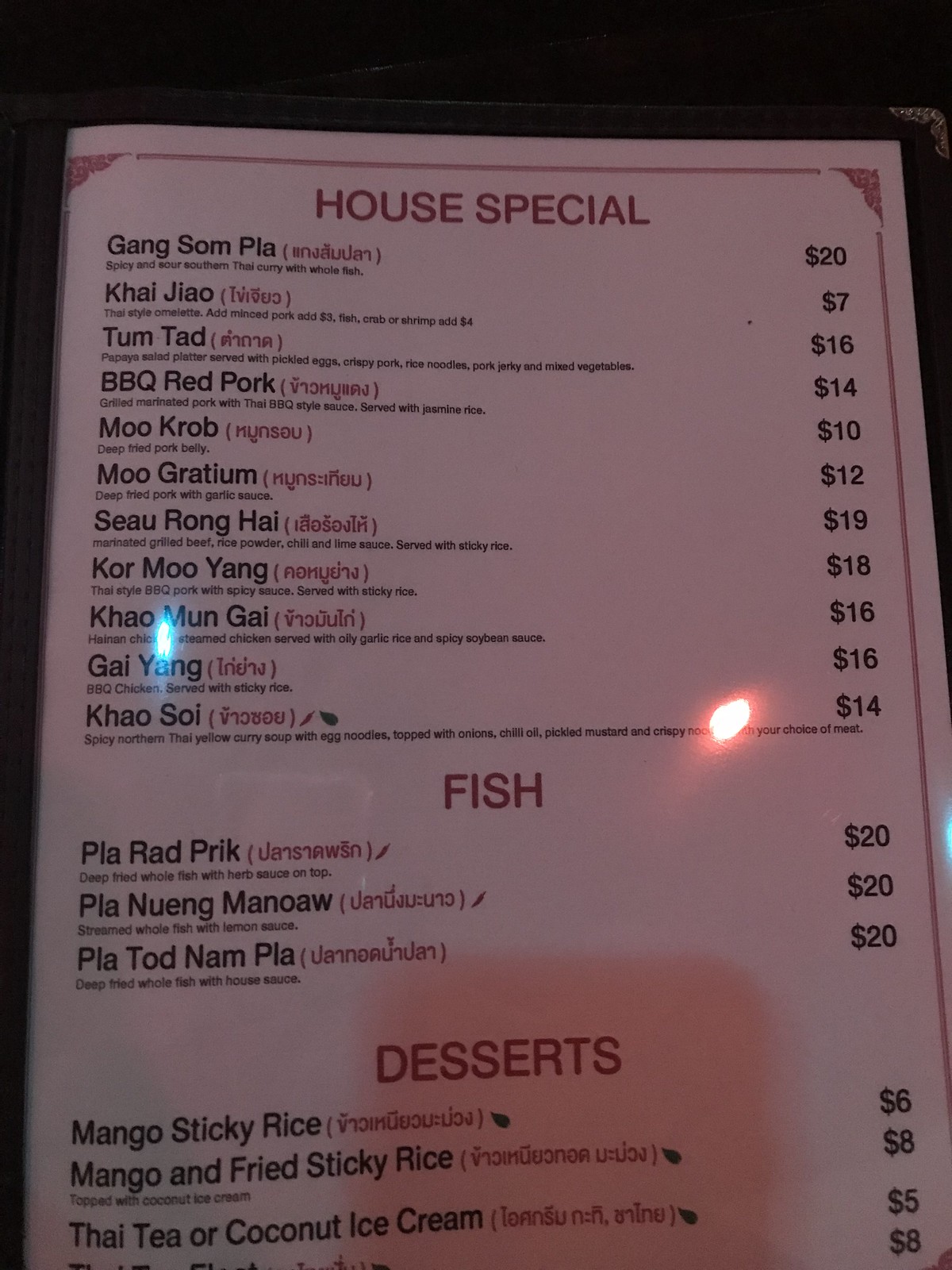The image portrays a menu set against a black background. The menu appears to be folded, evidenced by the noticeable red border descending along the right side, while the left side shows minimal visibility of this border. The corners of the menu highlight shaded-in red triangles. The primary focus of the menu is on the "House Specials," which feature a variety of dishes that can be considered a bit pricey for a Chinese restaurant. The listed items include Gangsam Pia, Cao Gio, Tom Tad, Barbecue Red Pork, Moo Crab, Moo Gradium, Shanrong Hall, Khor Moo Yang, Khao Mun Gai, Gai Yang, Khao So, Pia Rad Prick, Plo Nguyen Manow, Pia Todd Nam Plow, Mango Sticky Rice, Mango and Fried Sticky Rice, and beverages such as Thai Tea or Coconut Ice Cream. The entrees are notably priced around $20, and desserts are marked at $5 each.